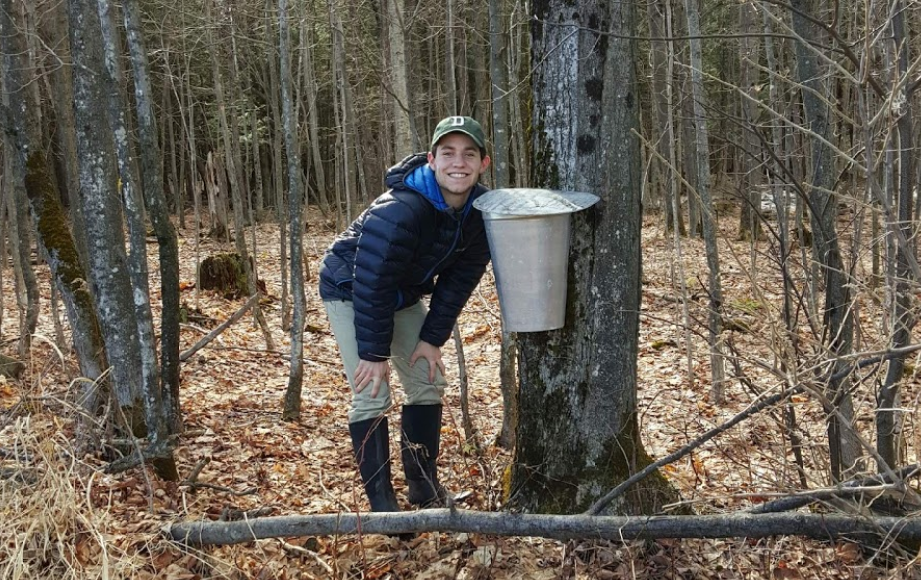The photograph, taken outdoors on a sunny day, captures a dynamic autumn scene in a forest scattered with dead brown and orange leaves. In the center of the image stands a thick, gray tree trunk adorned with a silver metal bucket used for gathering sap, protected by a flat round lid. Beside the tree, a young boy, approximately 12 or 13 years old of Caucasian descent, is crouched down. He sports a green baseball cap with a prominent 'D,' a navy blue puffer jacket with a light blue interior, light gray pants, and black rubber boots. With his hands braced on his knees, he leans towards the sap-gathering bucket, smiling happily at the camera, fully immersed in the syrup collecting process. The forest around him features barren tree branches and scattered shrubbery, enriching the rustic atmosphere likely indicative of a New England setting.